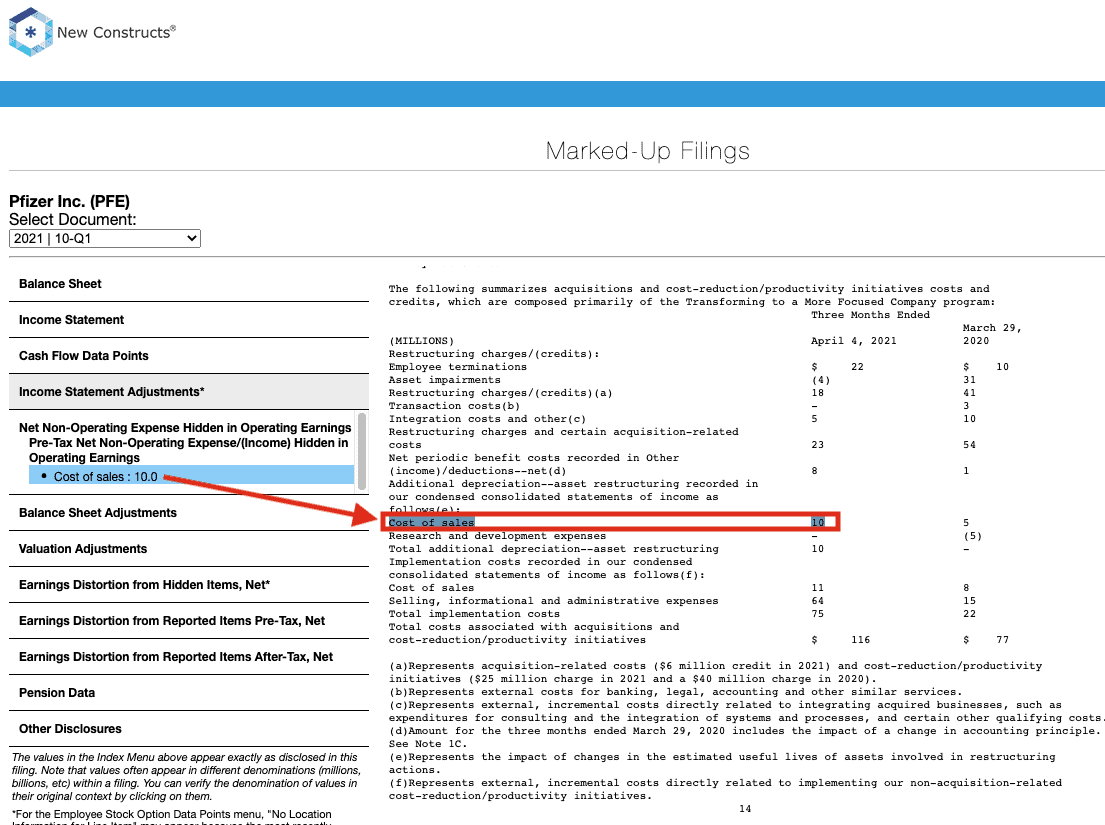Screenshot from "New Constructs" Documentation System: 

The image is a screenshot captured from a documentation system titled "New Constructs." At the top, a logo with the text "New Constructs" is prominently displayed, accompanied by a decorative blue line. Below the logo, the main title "Marked Up Filings" is centered.

Immediately beneath the title, there's a subheading, "Pfizer, Inc., PFE," paired with a drop-down menu labeled "Select Document," allowing users to navigate through various documents available for review.

On the left side of the interface, a vertical menu lists numerous options for financial documents and data points. This menu includes:

- Balance Sheet
- Income Statement
- Cash Flow Data Points
- Income Statement Adjustments
- Net Non-Operating Expense, Hidden in Operating Earnings
- Pre-Tax Net Non-Operating Expense Income, Hidden in Operating Earnings
- Balance Sheet Adjustments
- Valuation Adjustments
- Various earnings-related items
- Pension Data
- Other disclosures

The current active selection seems to be "Net Non-Operating Expense, Hidden in Operating Earnings," directing the viewer’s focus to specific financial details. 

On the right side of the screenshot, detailed financial data is displayed, with a particular emphasis on the "Cost of Sales" figure, noted to be 10. This section elaborates on various income-related metrics associated with the selected document, offering intricate insights into the financial performance of Pfizer, Inc.